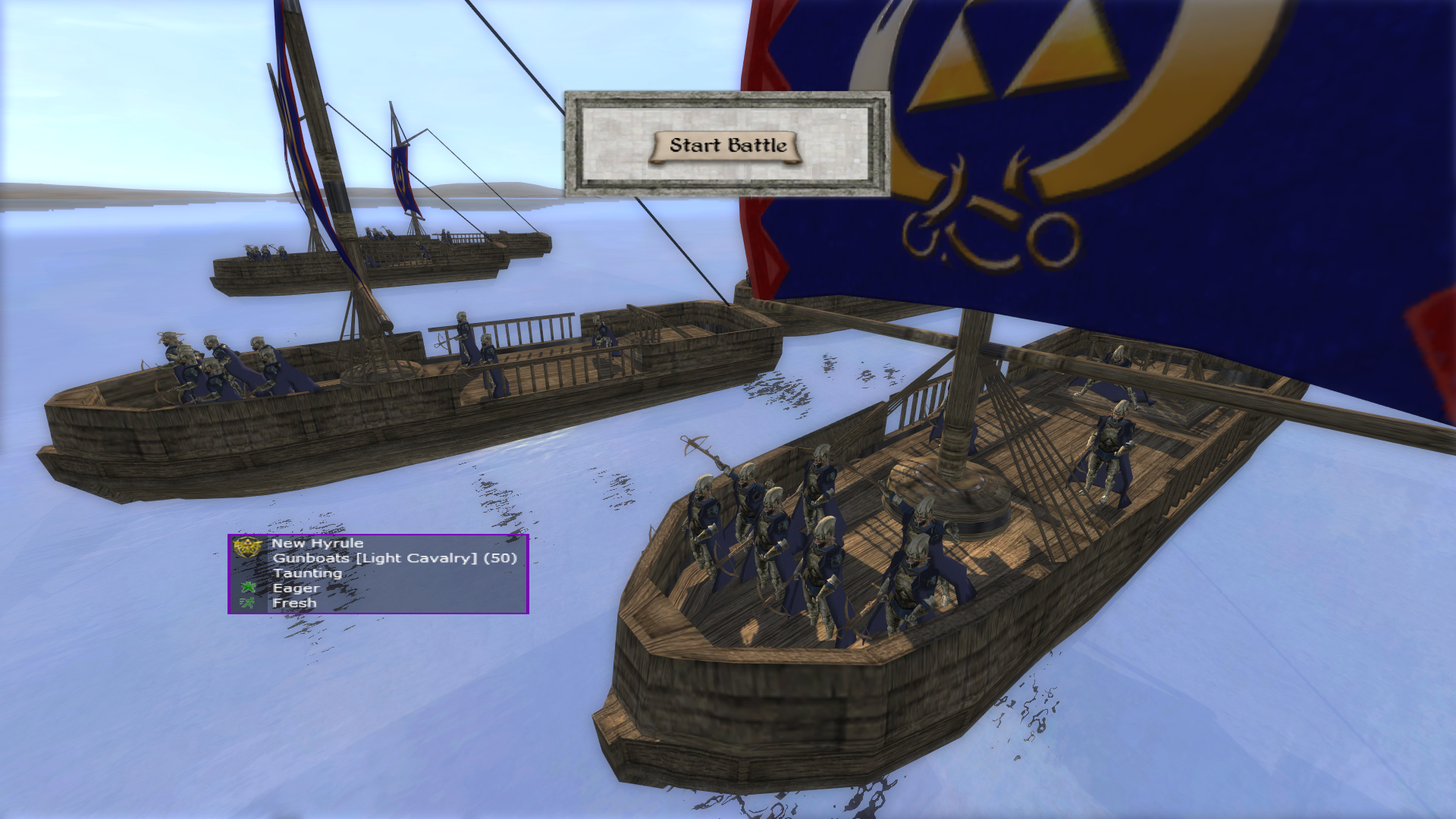The colorful screenshot from the game, likely related to the Legend of Zelda series, features a fleet of three old-fashioned ships with large sails. These ships are depicted with intricate details showcasing their wooden masts and deck setups, complete with shelters and cannons. The sails are adorned with the iconic Triforce logo, set against a blue background with golden accents. 

In the middle of the image, a parchment-like modal prominently displays the prompt "Start Battle," indicating the beginning of a naval confrontation. The bottom left corner of the screenshot highlights a key or legend that reads "New Hyrule Gunboats," followed by descriptors like "Light Cavalry 50," "Taunting," "Logger," and "Fresh." 

The ships are reminiscent of old exploration vessels, such as those used by Columbus, yet are distinct in their Zelda-themed design. Some sailors, possibly wearing blue capes and armor while wielding crossbows, are visible on the decks, prepared for action. Additionally, crates of unknown contents are scattered around. The scene captures a moment where one ship's sails are fully unfurled while the others appear to be in the process of setting sail, adding to the dynamic anticipation of the upcoming battle.